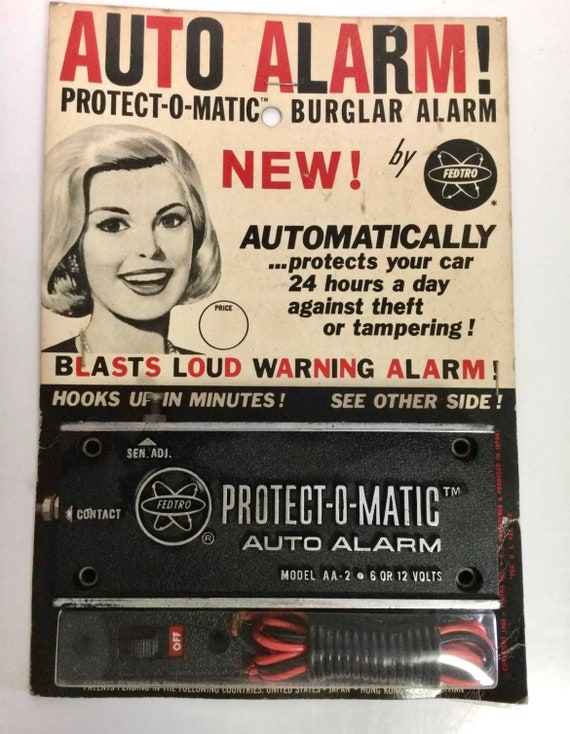This classic 1950s advertisement poster promotes the new Protect-O-Matic Auto Alarm by Fedro. The top half of the poster features yellowed, retro-style paper with bold, alternating red and black block letters proclaiming "Auto Alarm!" and "Protect-O-Matic Burglar Alarm," along with a note that it's a new product. A key feature of the ad is a smiling blonde woman with a 1950s hairstyle, suggesting ease of use. The text promises that the alarm "Automatically protects your car 24 hours a day against theft or tampering" and "Blasts a loud warning alarm." Below, text in black and red states that the device "Hooks up in minutes," with a prompt to "See other side." The lower section of the package, in black with a transparent plastic cover, showcases the alarm itself: the Protect-O-Matic Auto Alarm, model AA2, compatible with six or twelve volts. Also visible are a bundle of black and red cords, a contact point for connecting the device, and a prominent red on-off switch. The overall design is enshrined in a hole-punched display, hinting at its past life hanging on hardware store racks.